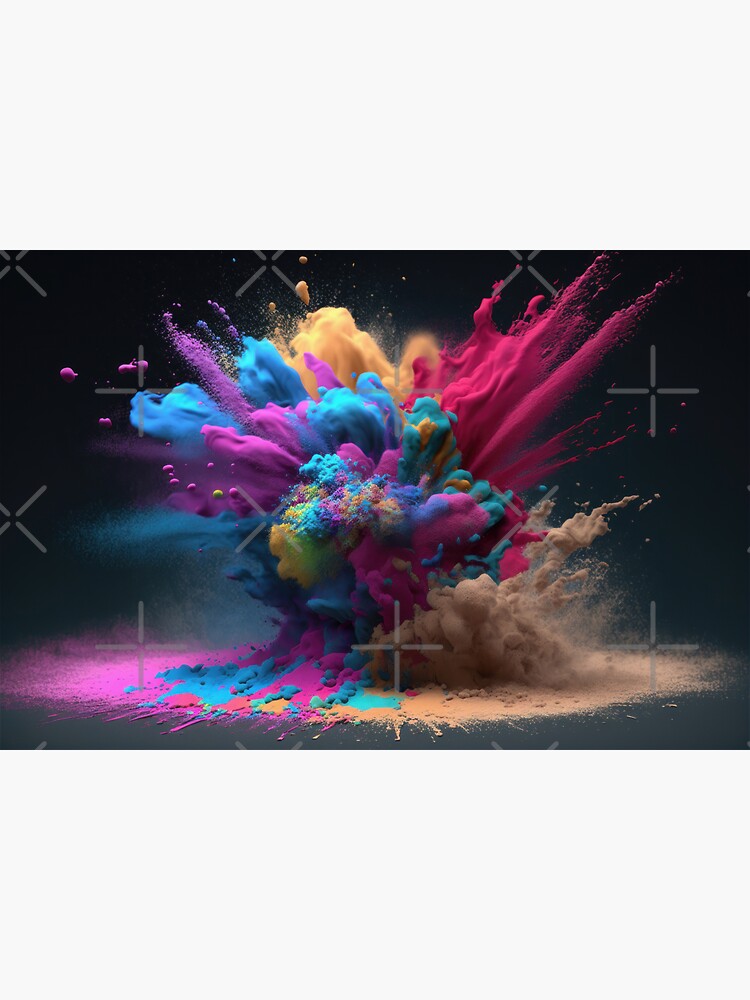This rectangular image features a central explosion of vividly colored sand and foam set against a black and slate-gray background, creating a smoky, 3D effect. The sides are framed by thick, light-gray headers and footers, each an inch in height, with the overall image measuring approximately six inches high and four inches wide. Transparent watermarks in the form of X's and pluses are scattered across the composition.

The scene resembles a vibrant, indoor artistic experiment, with a floor painted a dark gray and walls a lighter gray. On the lower right, brownish foam rises from the ground, while dark pink foam, almost sand-like in texture, covers the lower left. As the explosion erupts in the middle, it releases an array of colors including blue, yellow, pink, purple, and green, forming a dynamic, cloud-like burst. The left side of the explosion features pastel shades reminiscent of cotton candy, primarily in purple and blue, transitioning to yellow and orange in the background, and culminating in a vibrant pink on the right. The base of the explosion reflects these colors, adding a visually cohesive ground element with pink, blue, and green hues mingling with the sand-like brown on the right.